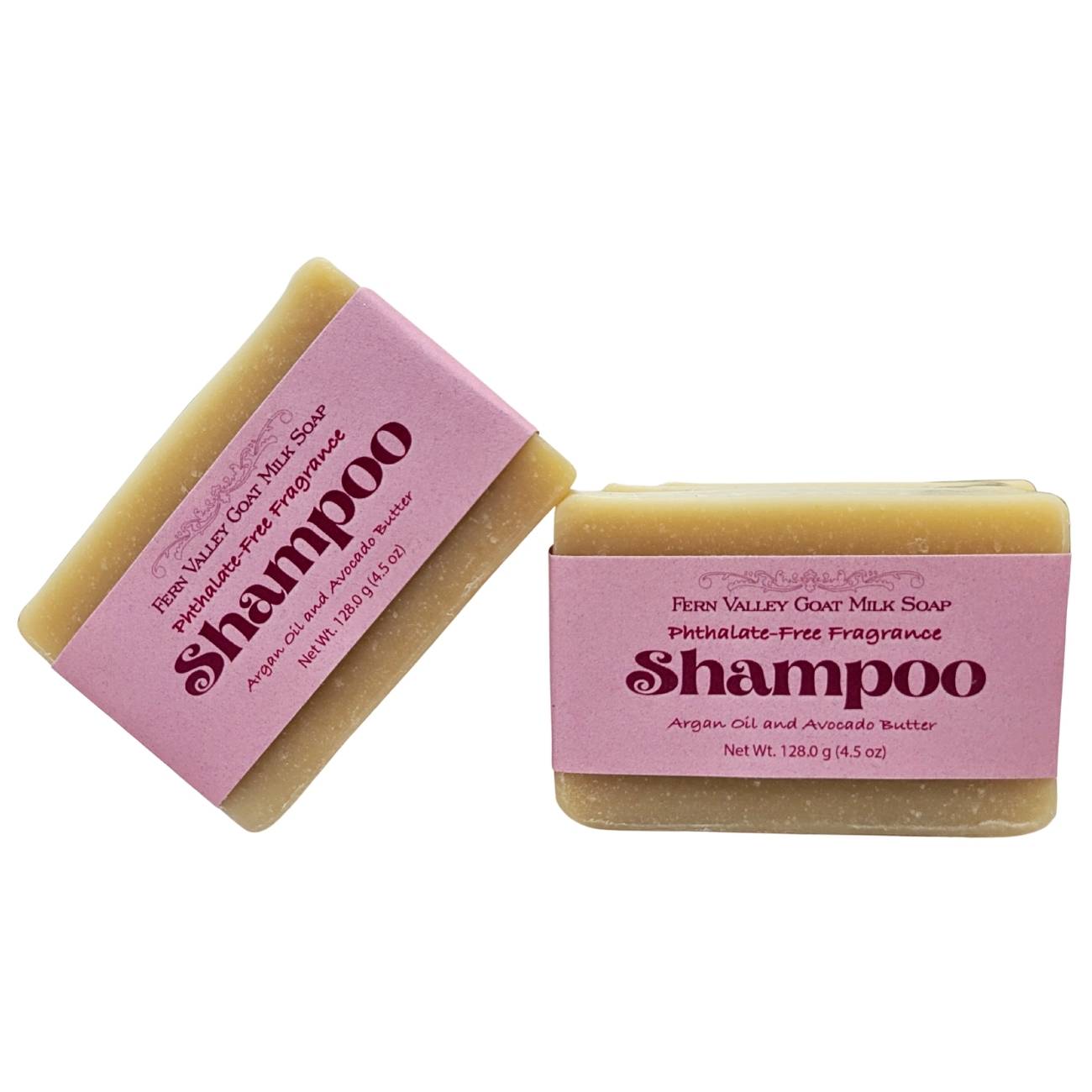The image showcases a pair of rectangular, porous bars of soap, each approximately two inches wide and one and a half inches high, set against a plain white background. The soap bars, which are a cream-tan color with flecks of cream, are adorned with pink cardboard bands featuring burgundy print. These bands are inscribed with "Fern Valley Goat Milk Soap" followed by "Phthalate-Free Fragrance Shampoo" in smaller text. Additionally, the labels specify that these shampoos contain Argan Oil and Avocado Butter, and each bar weighs 128.0 grams (4.5 ounces). The bar on the right is positioned upright, directly facing the viewer, while the bar on the left is tilted upward, resting its right half on the upper left corner of the right bar.